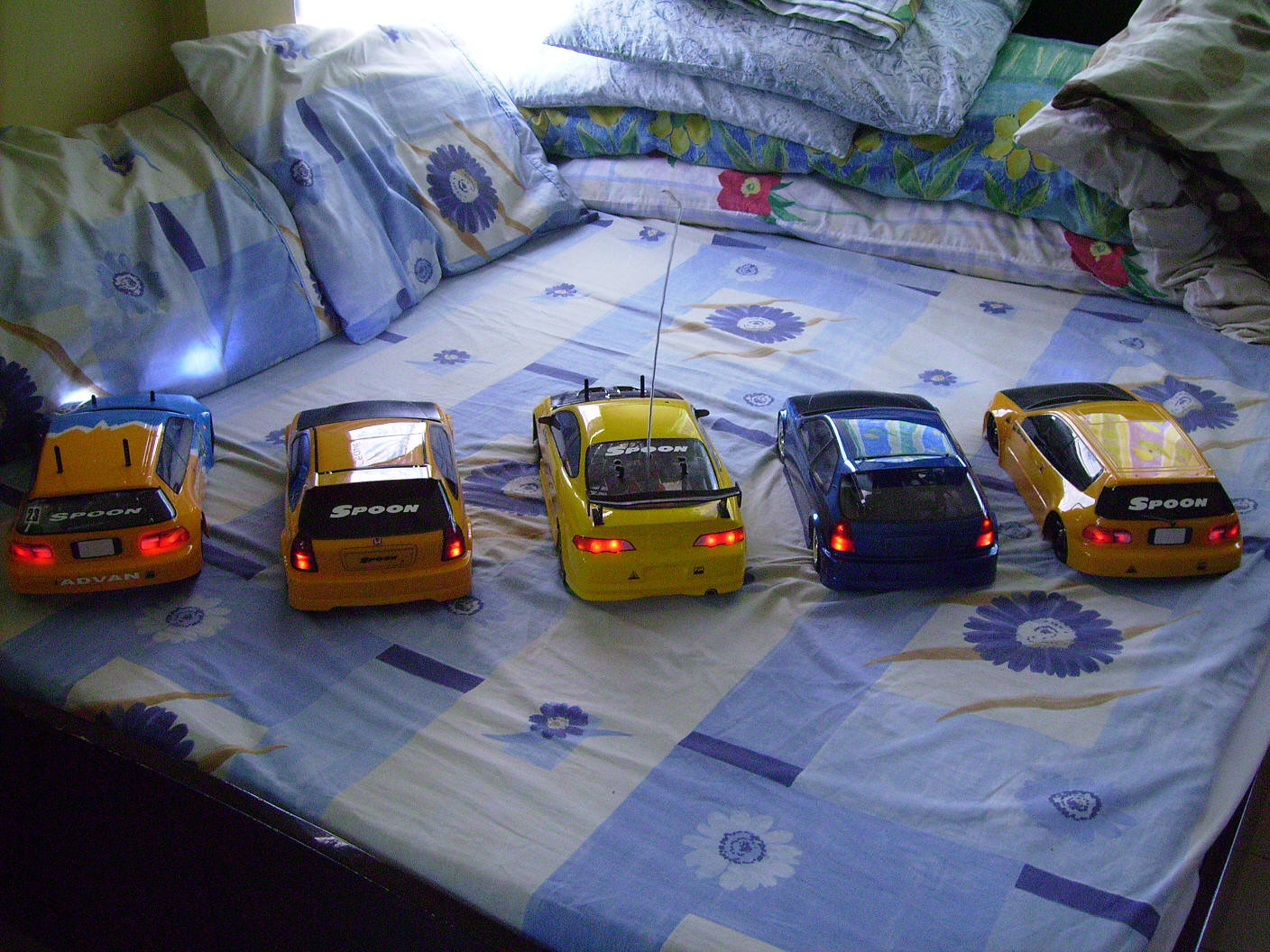This photograph captures a detailed scene of a bed adorned with multiple pillows and blankets, hosting a lineup of five model cars. The bed, which appears to be a queen or full-size, features a neatly tucked-in bed sheet with a design of blue and white stripes, complemented by blue and floral pattern pillows at the top. There are additional decorative pillows and two comforters stacked tidily on the right side of the bed.

Central to the image are five hatchback model cars, intricately displayed diagonally across the bedspread. These cars, detailed with illuminated brake lights and headlights, include three nearly identical orange hatchbacks, each bearing the text "SPOON" on their back windows. Positioned between the orange cars, there's a distinct yellow hatchback with a prominent long antenna and also marked with "SPOON," and a blue hatchback.

The room is lit by natural sunlight, casting subtle shadows over the bed, emphasizing the vibrant colors of the cars and the cozy, slightly wrinkled fabric of the bedding. This thoughtful arrangement of elements showcases both the intricacy of the model cars and the comfortable ambiance of the bedroom setting.